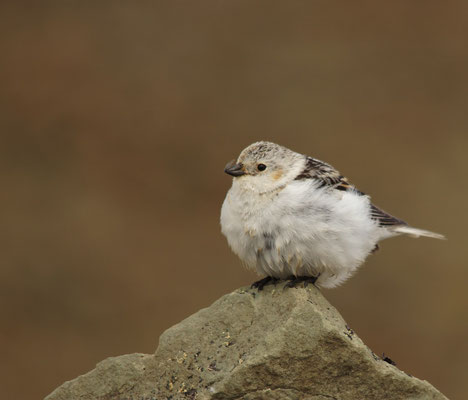The square-shaped image features a small, round, and plump bird perched atop the pinnacle of a naturally-formed, triangular gray rock situated at the bottom middle edge of the frame. Facing roughly the seven or eight o'clock direction (leftward), the bird is characterized by its light grayish-white chest and breast feathers, speckled light-colored head, and darker gray and black markings on its back and wings. The tiny creature has a stout head with short gray hair, black beady eyes, a small black beak, and black feet. A distinct longer white tail feather extends behind the bird, which appears stationary and not in motion. The background is blurred with neutral tones of brown and gray, adding a natural and serene ambiance to the image.